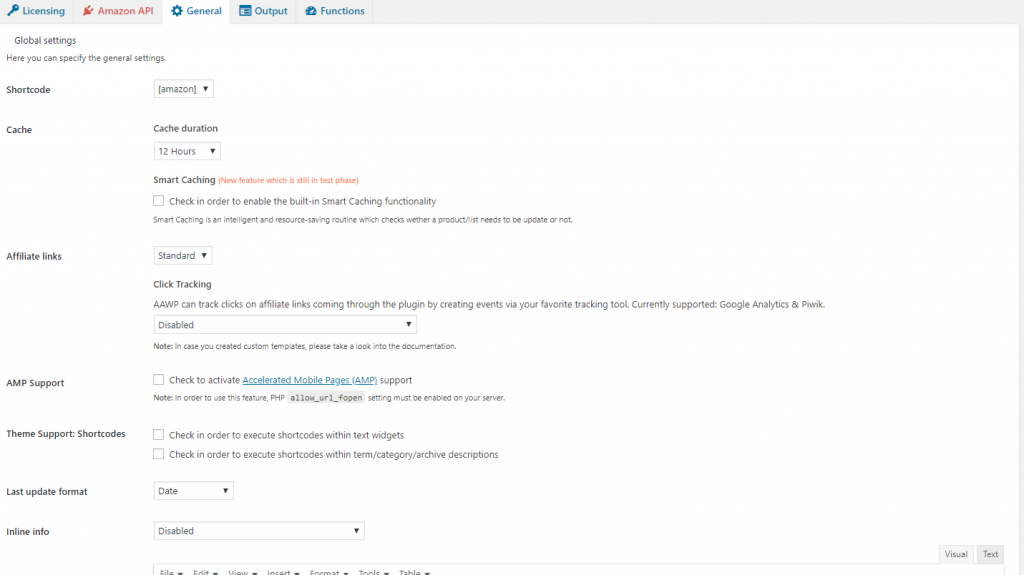This image depicts an online form interface, specifically for Amazon settings. The upper left corner features multiple tabs, including "Licenings," "Amazon API," "General Settings," "Output," and "Functions," with the "General Settings" tab currently active. The "General Settings" page displays a section titled "Global Settings" on the left, where users can configure various options. The settings listed include "Shortcode," "Affiliate Links," "Cache," "AMP Support," "Theme Support Shortcodes," "Last Update Format," and "Inline Info." The main area of the form contains several input bars and checkboxes for each configuration option. The interface has a clean, white background, enhancing readability and user navigation.